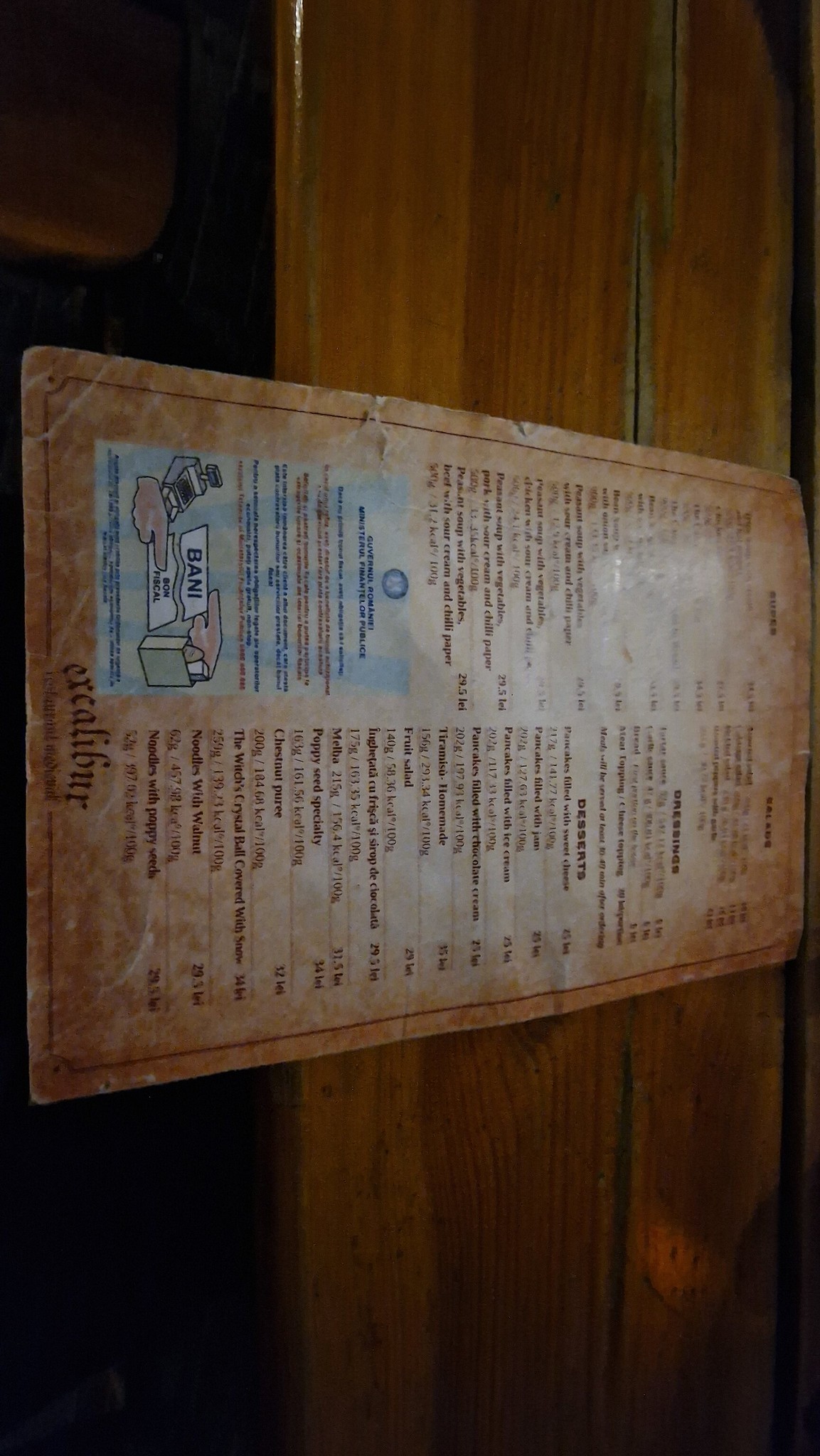In this photograph, a vintage menu is prominently displayed. Although the image is taken from a landscape perspective, the menu is oriented upright as if standing, though it actually lies flat on a wooden table. The menu is discolored, presenting a brown, textured appearance that accentuates its aged look. The text on the menu is in two different languages, with headings such as "Souffle," "Dressings," and "Desserts" appearing in an elegant, old-fashioned font. A distinctive blue square with minimal text and blue-striped detailing provides a striking contrast to the overall sepia-toned design. The graphic elements are minimal, focusing primarily on the text and accompanying prices. The wooden surface on which the menu rests adds to the rustic, nostalgic ambiance of the scene.